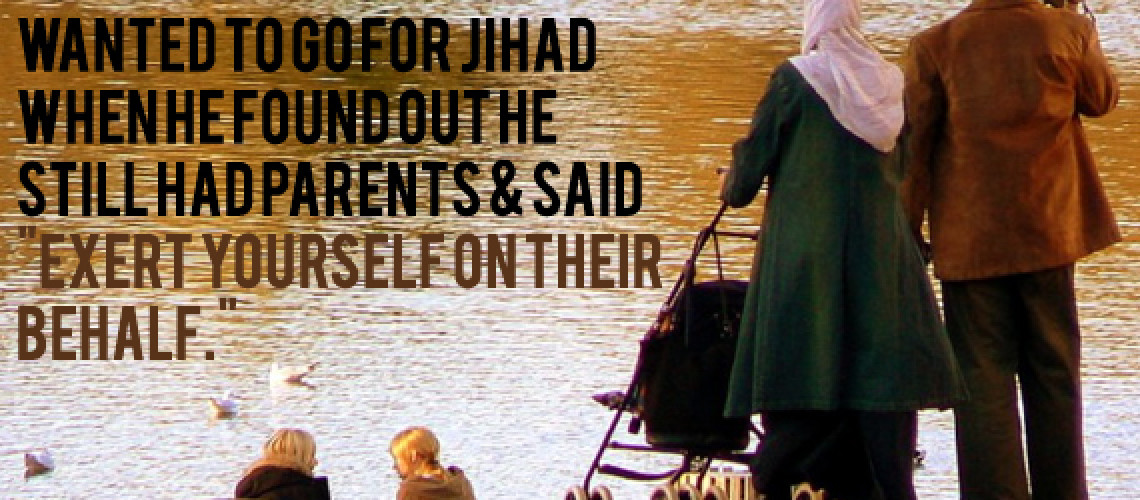The image is a card featuring a photo set against a background of murky, brown water, likely a river or lake. In the lower-left corner, the shoulders-up profiles of two blonde individuals, presumably children, are facing each other, engaged in conversation. They are depicted sitting by the water. In the foreground on the right, a Muslim woman wearing a green coat, dark pants, and a pinkish-white head covering extends her left arm, holding onto a stroller. To her left stands a man dressed in a rusty-colored coat and dark brown pants, with his head cropped out of the frame. The left half of the card is dominated by large text. In black, it reads, "wanted to go for jihad when he found out he still had parents." Below, in brown letters, it says, "exert yourself on their behalf." Scattered across the water are white seagulls, adding further depth to the serene yet melancholic setting.